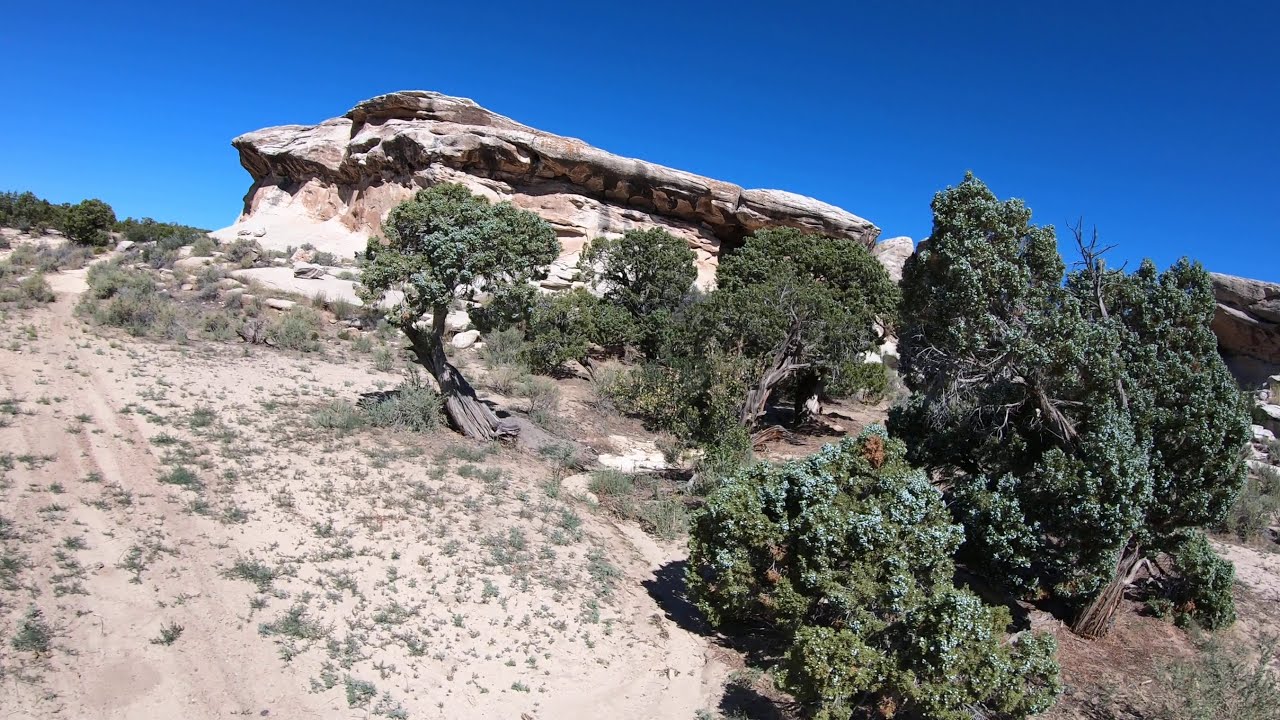This image captures a remote, wild hillside landscape bathed in bright sunlight under a deep, vibrant blue sky. The scene looks up a dusty, grassy hill, featuring patches of vegetation interspersed with dry, tan dirt. On the left side, small green patches frame the path, while on the right, stubby trees with dark green, somewhat dried-up leaves ascend the slope. The trees are fairly short and sparse, providing little shade and not obstructing the sky.

Dominating the upper part of the hill is a large, rocky outcropping or plateau that extends laterally, adorned with shades of pale coral, gray, and cream. Beyond this rocky feature, a more forested area is suggested by additional short trees. The landscape also shows a sandy path winding up from the bottom left, marked by visible tracks, possibly from an all-terrain vehicle. Overall, the image conveys a sense of dry, rugged terrain highlighted by nature's raw and untamed beauty, devoid of clouds and framed by the intense blue sky.